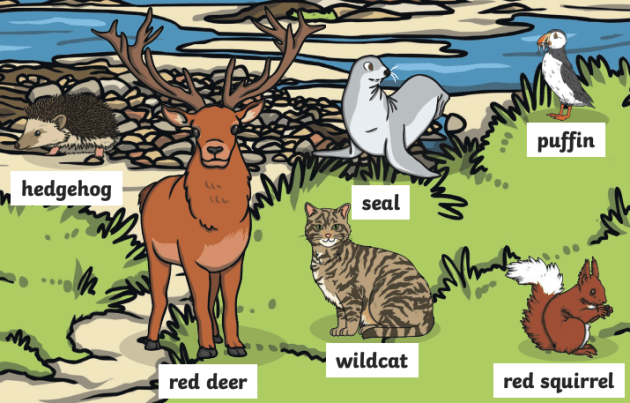This image is a detailed illustration showcasing various animals typically found in a forest setting, rendered through a mix of painting and drawing techniques. The scene is lush and vibrant, featuring green grass at the bottom, a water area at the top, and several stones situated between the two. The animals are organized into two rows: on the top row from left to right, there is a hedgehog, a seal, and a puffin. The bottom row, also from left to right, includes a red deer, a wildcat, and a red squirrel. Each animal is depicted in a distinctive color palette: the red deer is in red, the wildcat in a blend of light and dark brown, and the red squirrel in red and white. Adjacent to each animal, there is a white rectangle containing the name of the animal written in black text. This illustration serves as an informative guide to the animals one might encounter in a specific type of nature setting, emphasising a forest environment with elements like grass, water, stones, and dirt.